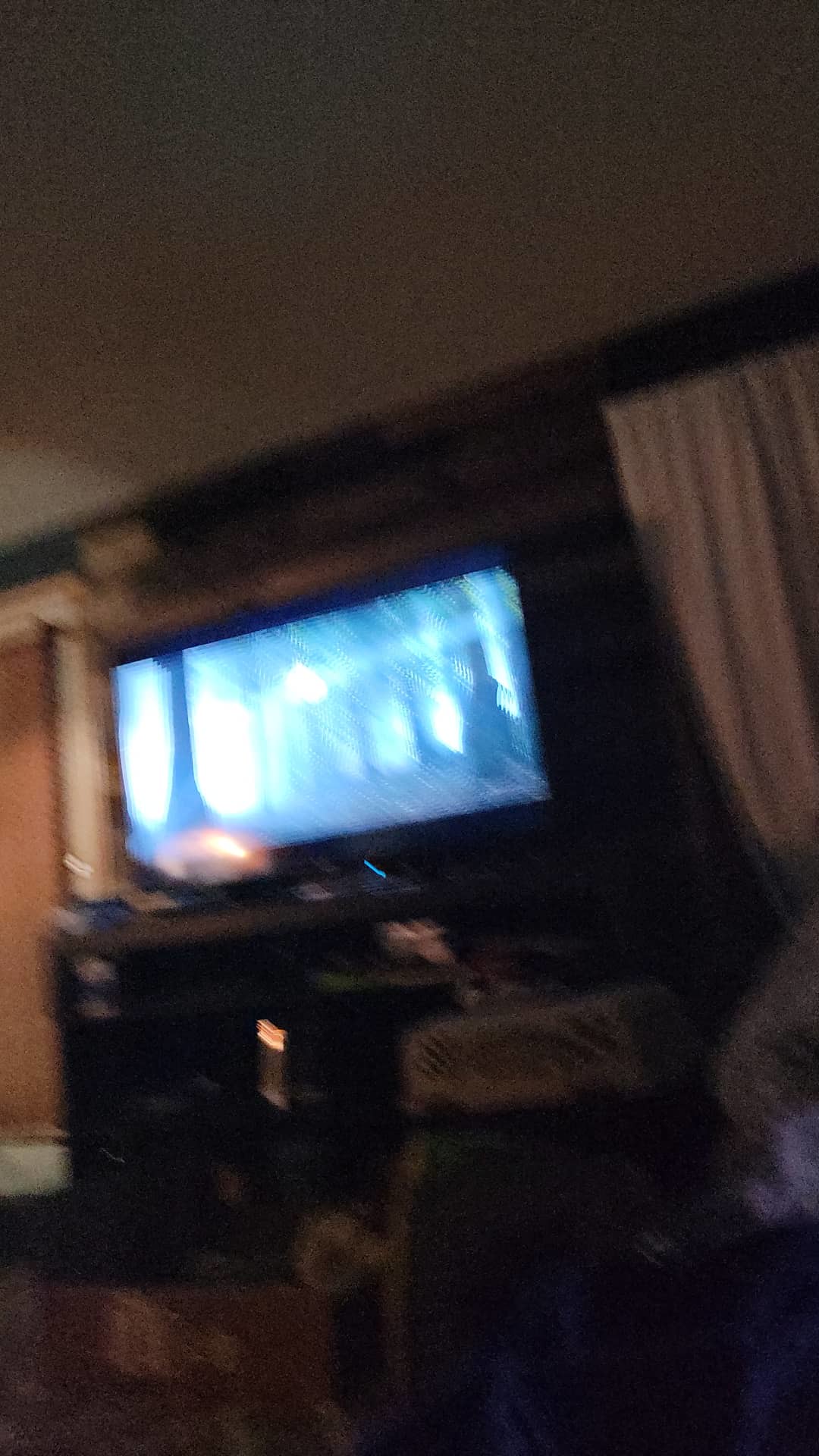The image captures an indoor scene marked by significant blurriness and low resolution. Despite the lack of clarity, certain elements are discernible. The center of the background features a rectangular TV, which is faintly displaying something indistinct, emitting a whitish light. Above, the ceiling is noticeable in a white hue. To the right of the TV, white-colored curtains are visible. The TV itself is positioned on some piece of furniture. The overall impression is one of motion and fuzziness, rendering the finer details obscure.